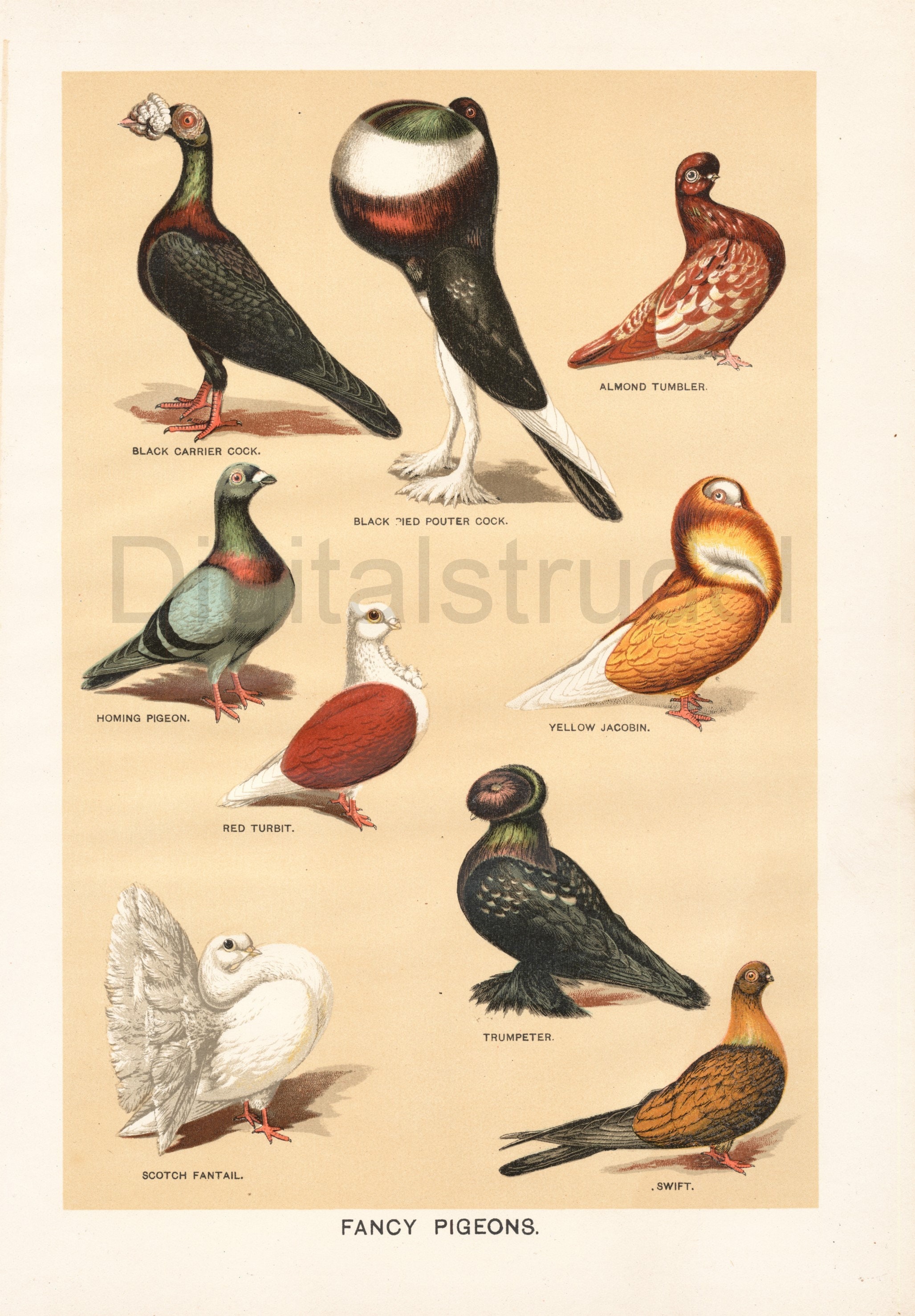The image depicts an educational poster titled "Fancy Pigeons," showcasing nine distinct pigeon breeds arranged in three rows of three. Set against a peach-beige background with a coral top border and an orange center, the poster highlights the unique characteristics of each bird. Starting from the top left, the Black Carrier Cock is identified by its dark feathers, red and green iridescence around its neck, and stark red eyes. Next is a Black Pied Pouter Cock, notable for its exaggerated, tennis ball-like crop and black feathers with a green-and-red sheen. The top row is completed by the Almond Tumbler, which has a striking red S-shaped body.

In the middle row, the Homing Pigeon sports a typical grey color with black tail stripes and a mix of reddish and greenish hues on its head. Beside it, the Red Turbot is predominantly white with a distinctive red oval patch on its wing. The Yellow Jacobin, on the far right, appears golden-brown with an ornate, scarf-like feather arrangement around its neck.

The bottom row begins with the Trumpeter, distinguishable by its circular head and vibrant purple, green, and black plumage. The Swift, found next, features a sleek brownish-golden color with a dark tail, and the row is concluded by the white Scotch Fantail, resembling a swan with its puffed-up rear feathers. This detailed poster not only educates but also visually celebrates the diverse and striking features of these fancy pigeon breeds.